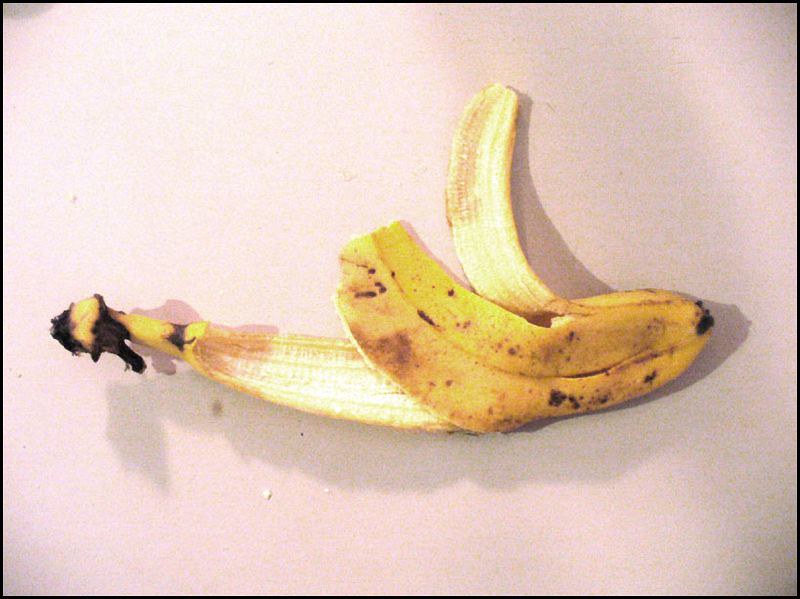The photograph captures a partially eaten banana resting on a subtly textured cloth with a pinkish hue, likely due to the lighting. The cloth features gentle folds and shadows, adding a sense of depth and softness to the background. The banana peel, predominantly brown and indicative of ripeness, stretches horizontally across the image. Inside the peel, approximately 25% of the remaining banana is visible, appearing very soft and slightly squashed. Scattered around the banana peel on the cloth are a few small bits of banana, contributing to the overall sense of casual disarray in the scene.